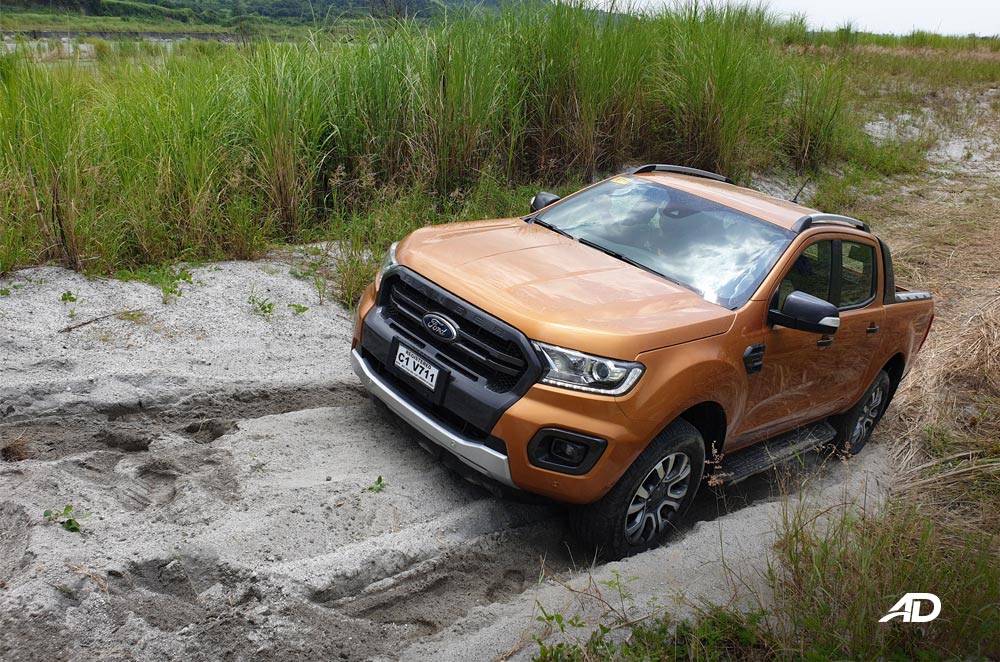In this photo, a new model Ford pickup truck, likely an Explorer or a Ranger, is depicted during an off-roading adventure in a marshy, muddy landscape. The truck, with a striking copper orange paintwork, features an extended cabin that comfortably seats four passengers and has a short truck bed. The vehicle is navigating over a gray, sandy, and muddy hill, with its black grill and white license plate (C1V711) clearly visible. The sandy ground underneath appears wet, indicating recent rains or marshland conditions, and the truck's tires are digging into the terrain. In the background, tall, light brown and green grasses typical of this marshland environment can be seen. To the upper left of the image, a grassy mountain range or hills stretch into the distance, while the upper right shows a white sky and green grass alongside a brown dirt road. The image, taken during the day, also has "AD" written in white in the bottom right corner, adding a subtle branding element.